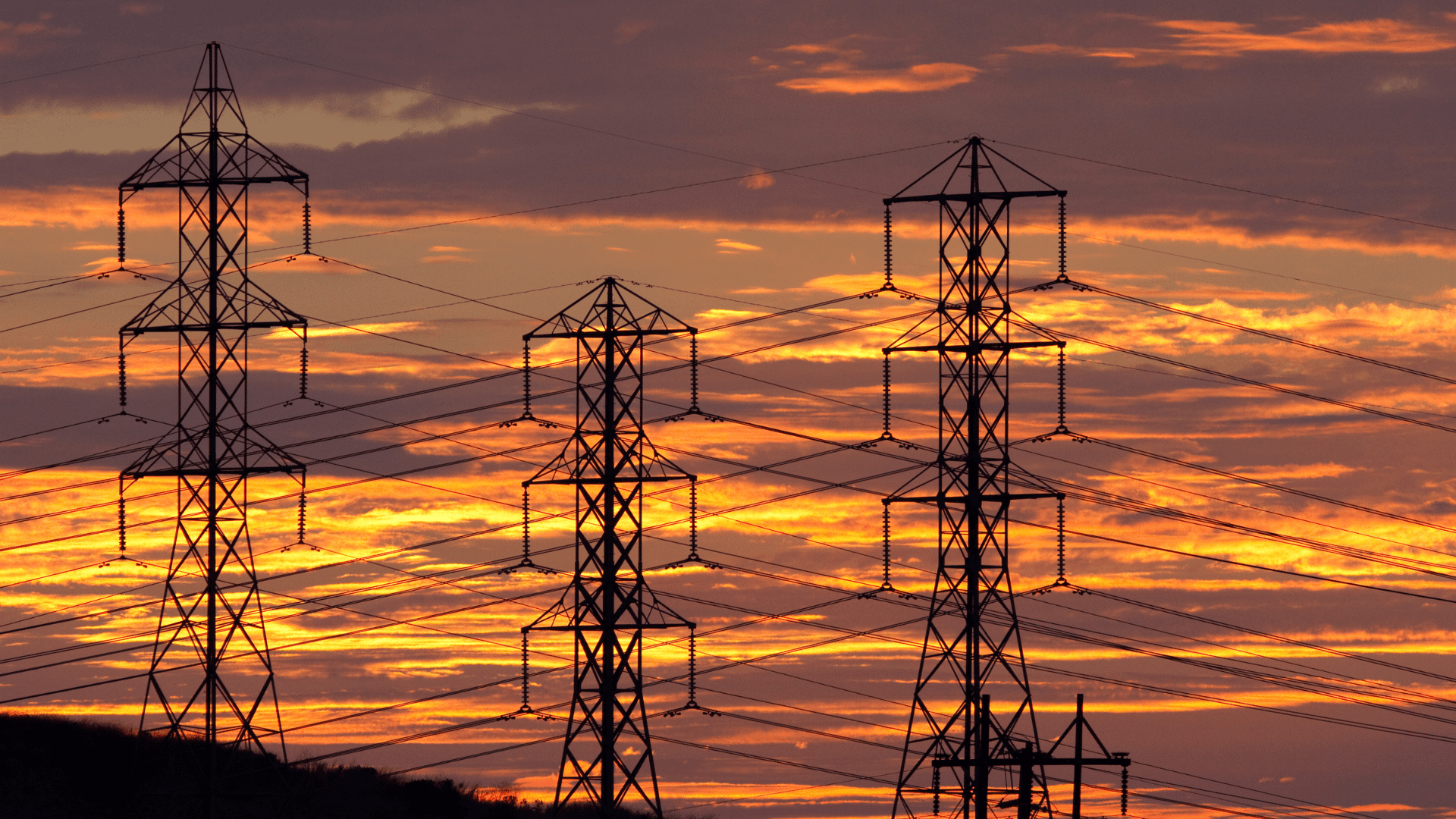This photograph, taken at either sunset or sunrise and painted in hues of orange, yellow, and pink, features three prominent electrical towers. These towering metal structures rise up into the sky, their lattice constructions visible against the backdrop of illuminated clouds. The towers are connected by a network of power lines, crisscrossing the image in multiple layers, each strand attached to jutting metal arms at various heights. On the left, the ground is visible but shrouded in deep shadows, revealing sparse greenery around the base of the leftmost tower. The middle tower stands slightly taller with minimal grass surrounding it, while the rightmost tower, also tall, appears devoid of any vegetation. The intricate web of electrical cables stretches across the entire photograph, weaving a complex pattern that punctuates the serene, colorful sky with industrial precision.